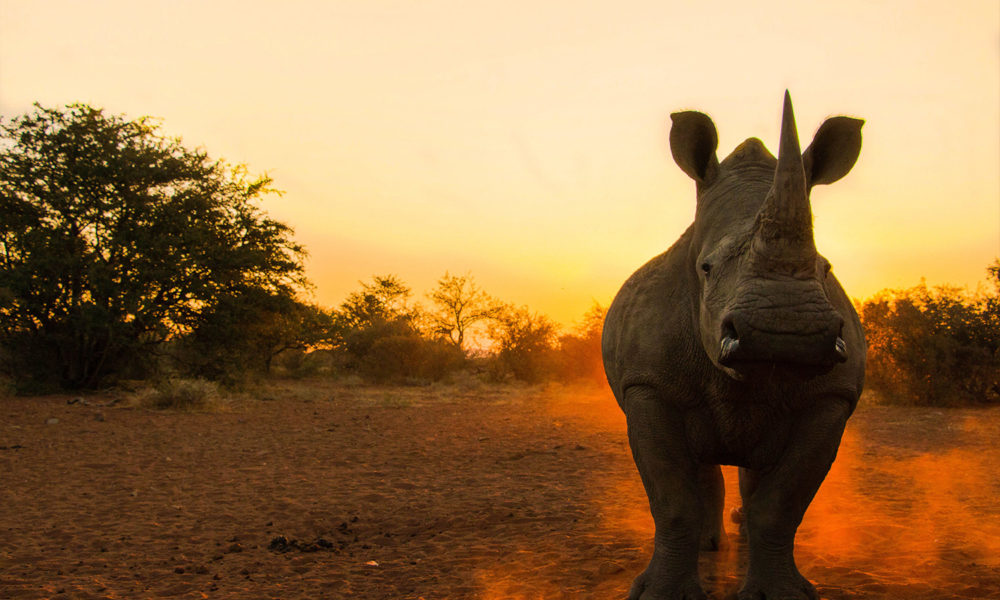The photograph captures an outdoor daylight scene featuring a majestic rhinoceros as the main subject, positioned prominently in the center-right foreground. The imposing animal has a single large upright horn above its nose, two expressive dark eyes, and small rounded ears that point to the sides of its head. It stands on a flat, dirt-covered ground, where it appears to be kicking up orange-hued dust that floats around its sturdy legs, possibly captured in motion or having just come to a stop.

The background reveals a transitional landscape with a series of scattered low trees and bushes, extending across a mildly elevated terrain. Notable is a large tree to the left, while smaller bushes are more dispersed toward the right. The sky overhead is awash with vibrant colors, transitioning from a golden brightness near the horizon to a paler yellow higher up, suggesting a low-hanging sun characteristic of either early morning or late evening, casting a soft, radiant glow over the scene. The overall atmosphere is one of serene natural beauty, highlighting both the ruggedness of the rhinoceros and the tranquil yet dynamic setting surrounding it.